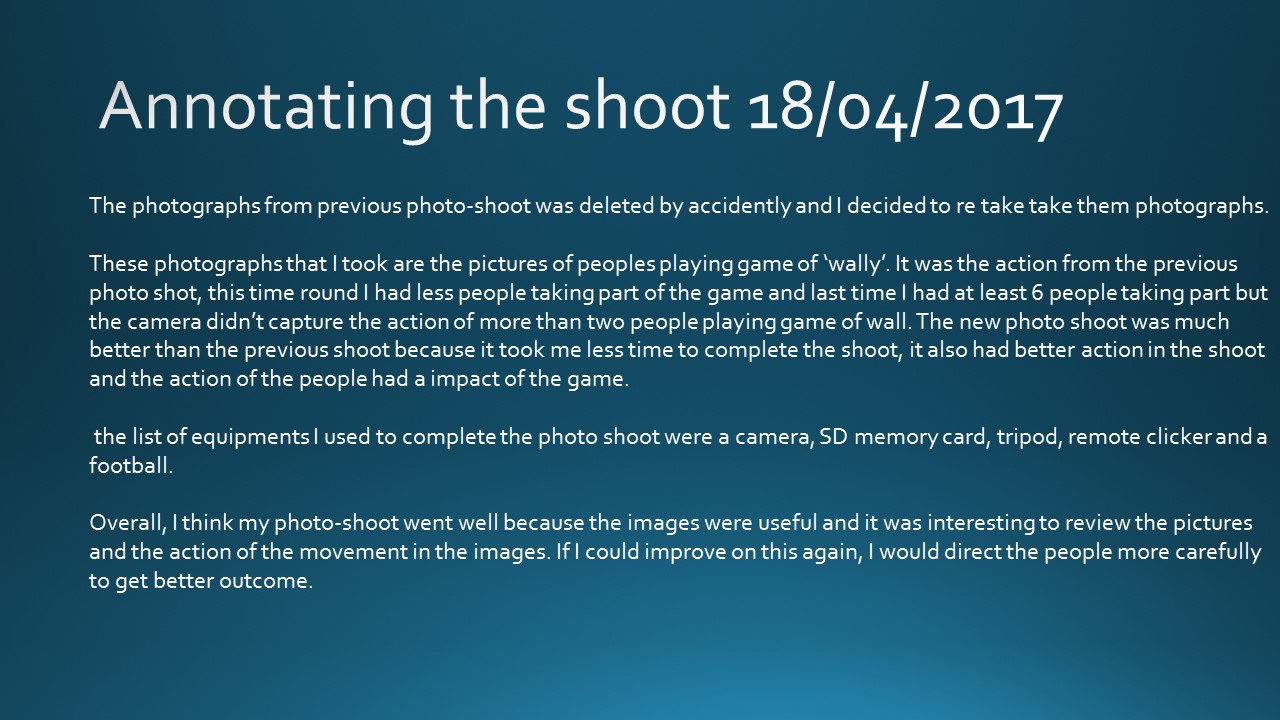The image is a PowerPoint slide with a dramatic gradient background that transitions from a shiny dark blue at the top to a lighter blue towards the bottom. At the top, large white text reads "Annotating the Shoot 18/04/2017". Below this, in smaller white font, the slide explains that the photographs from a previous photo shoot were accidentally deleted, prompting a re-shoot. The text goes on to detail the new photographs, which capture people playing a game of Wall. The creator notes that unlike the previous shoot involving six participants, this time only two people's actions were captured, though the overall quality of the photo shoot improved. The equipment listed includes a camera, SD memory card, tripod, remote clicker, and a football. Reflecting on the process, the photographer believes the images were useful and interesting, but notes that more careful direction of participants could lead to an even better outcome.